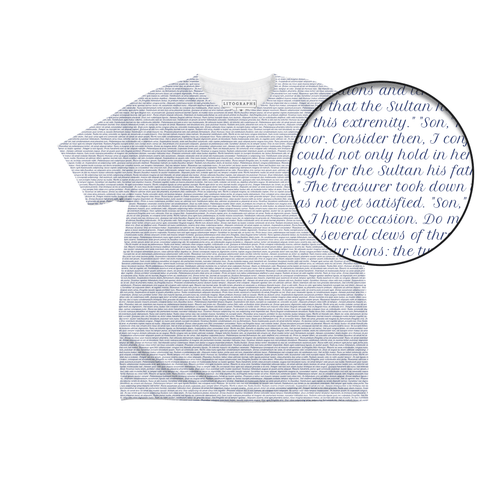This image depicts a gray, cotton, crew neck t-shirt meticulously laid flat on a white background, seemingly a child's size. Though appearing plain at first glance, an inset circle magnifies an intriguing detail on the right shoulder extending towards the upper left portion. This zoomed-in section reveals a dense lithographic pattern comprised of gray-printed words, including "sultan," "treasure," and "occasion," suggesting an inspirational or narrative theme. The t-shirt features a tagless design, with the label printed directly onto the fabric for added comfort.